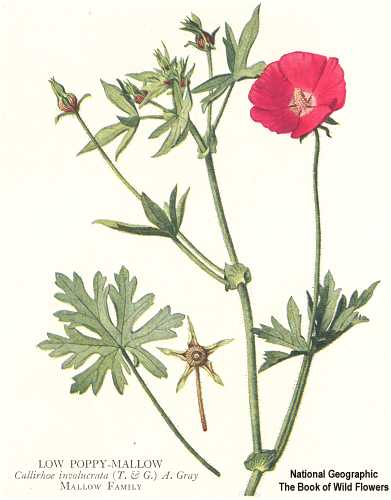The hyper-realistic drawing, featured in National Geographic's "The Book of Wildflowers," depicts a vibrant low poppy mallow (Kaliro involucrata). At the forefront of the image is a single red blossom with a few delicate petals, while multiple green stems extend upward, adorned with serrated leaves. A prominent leaf is positioned to the right, and a cluster of unopened buds occupies the upper section, hinting at forthcoming blooms. The detailed illustration includes text on the lower left, identifying the flower with its common and scientific names, along with the family classification. The beige background enhances the botanical details, making the intricate flower study appear lifelike.